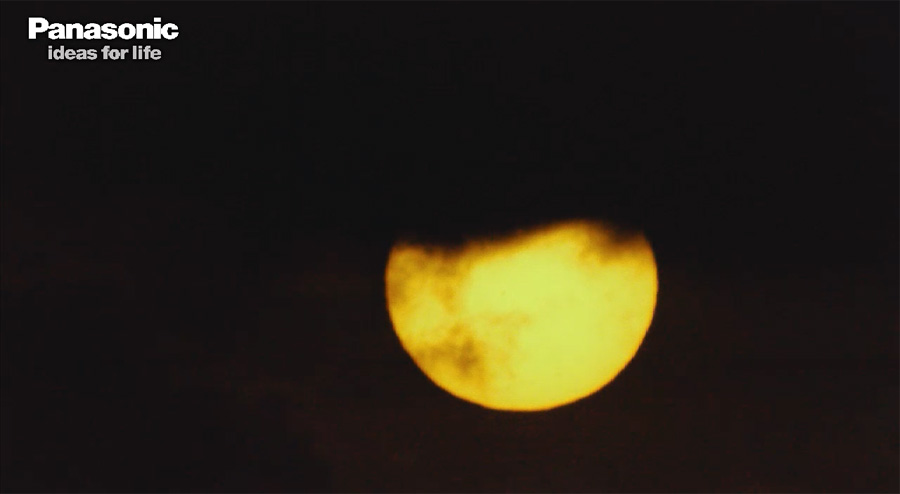The photograph, seemingly captured through a telescope, showcases a slightly blurry, glowing yellow circle that resembles the sun. This circle, positioned slightly to the right and lower in the frame, is partially obscured at the top by what appears to be a dense, dark smog or cloud-like formation. The dark areas of smog add a textured, shadowy quality to the vibrant yellow surface, set against an almost pitch-black background. The image's aspect ratio is slightly longer and narrower than typical photographs. In the upper left corner, the text "Panasonic" appears in crisp white letters, followed by the slogan "Ideas for Life" in a lighter gray font.